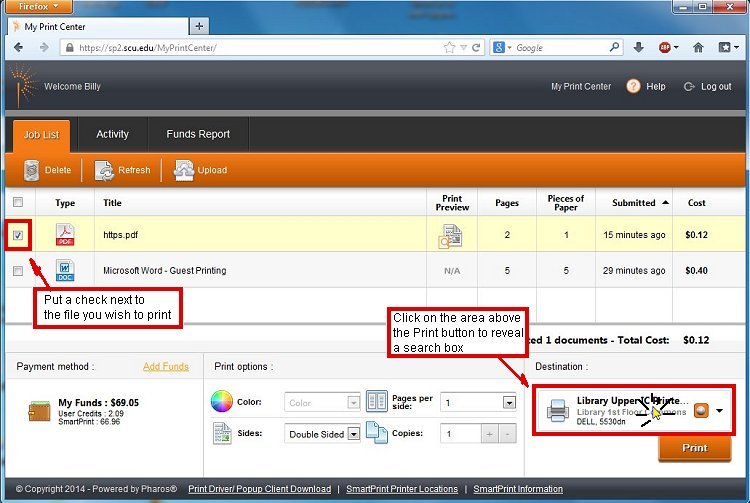The image is a screenshot of a computer screen displaying the Firefox web browser. The sole open browser tab is titled "My Print Center." In the address bar, the URL reads "https://sp2.scu.edu/MyPrintCenter/". In the top navigation bar, on the left-hand side, there is a logo resembling a sparkler, alongside the greeting "Welcome Billy." On the right side of the bar, it displays "My Print Center" along with "Help" and "Logout" buttons.

Beneath the top bar, three tabs are visible: "Job List" (the currently active tab), "Activity," and "Funds Report." Inside the "Job List" tab, there are options to "Delete," "Refresh," or "Upload." Overlaid on the screen are instructions explaining the functionality of the Print Center website. A PDF document is listed in the job queue, with a note indicating "put a check next to the file you wish to print." Additional instructions mention clicking an area above the print button to reveal a search box.

Further down, the interface displays a funds list in the payment method section, showing the available balance. Various print options are available, such as selecting color, number of sides, pages per side, and number of copies. In the bottom right-hand corner, there is a prominent orange "Print" button.